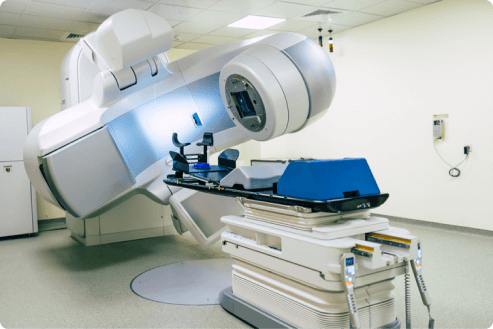The image showcases a sophisticated, expansive medical lab featuring a colossal scanning machine, likely an advanced MRI or CT scanner. Central to the scene is a gurney-style patient bed adorned with blue and gray pads, complete with a black headrest and devices for supporting legs. This bed is intricately connected to the massive, rotating scanning apparatus equipped with a substantial imaging camera capable of multiple-directional movement, possibly up to 360 degrees. The machine's structure is imposing and appears to emit light from its center, enhancing its mechanical and futuristic appearance. In the background, a white cabinet that resembles a refrigerator can be seen, alongside an arrangement of wires or tubing affixed to the right wall. The room is lit by a suspended ceiling with white rectangular lights, contributing to the clinical ambiance of the setting.